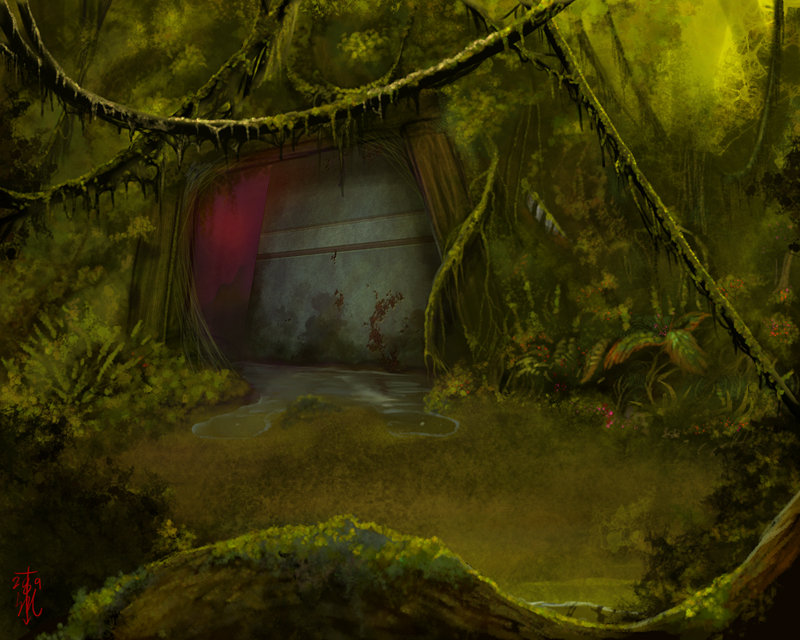This dark, jungle-themed illustration showcases a mysterious entranceway partially concealed by lush greenery. The scene is dominated by deep green and black tones, with a slight illumination from above. The main feature is a trapezoid-shaped door embedded into a stone wall, with the right side of the door being more sharply diagonal compared to the almost straight left side. The door is composed of three main sections: a vertical red strip on the left, a top half section that appears weathered and clings to the stone, and a bottom portion divided by a thin bar, marked by wet, red spots. Surrounding the entrance are thick jungle vines and a moss-covered tree branch extending from the bottom left corner to the center, then down to the bottom right. The stone landing in front of the door contrasts with the surrounding lush, yet wilting, vegetation and a dark green pond, enhancing the eerie ambiance typical of a cinematic or video game environment.